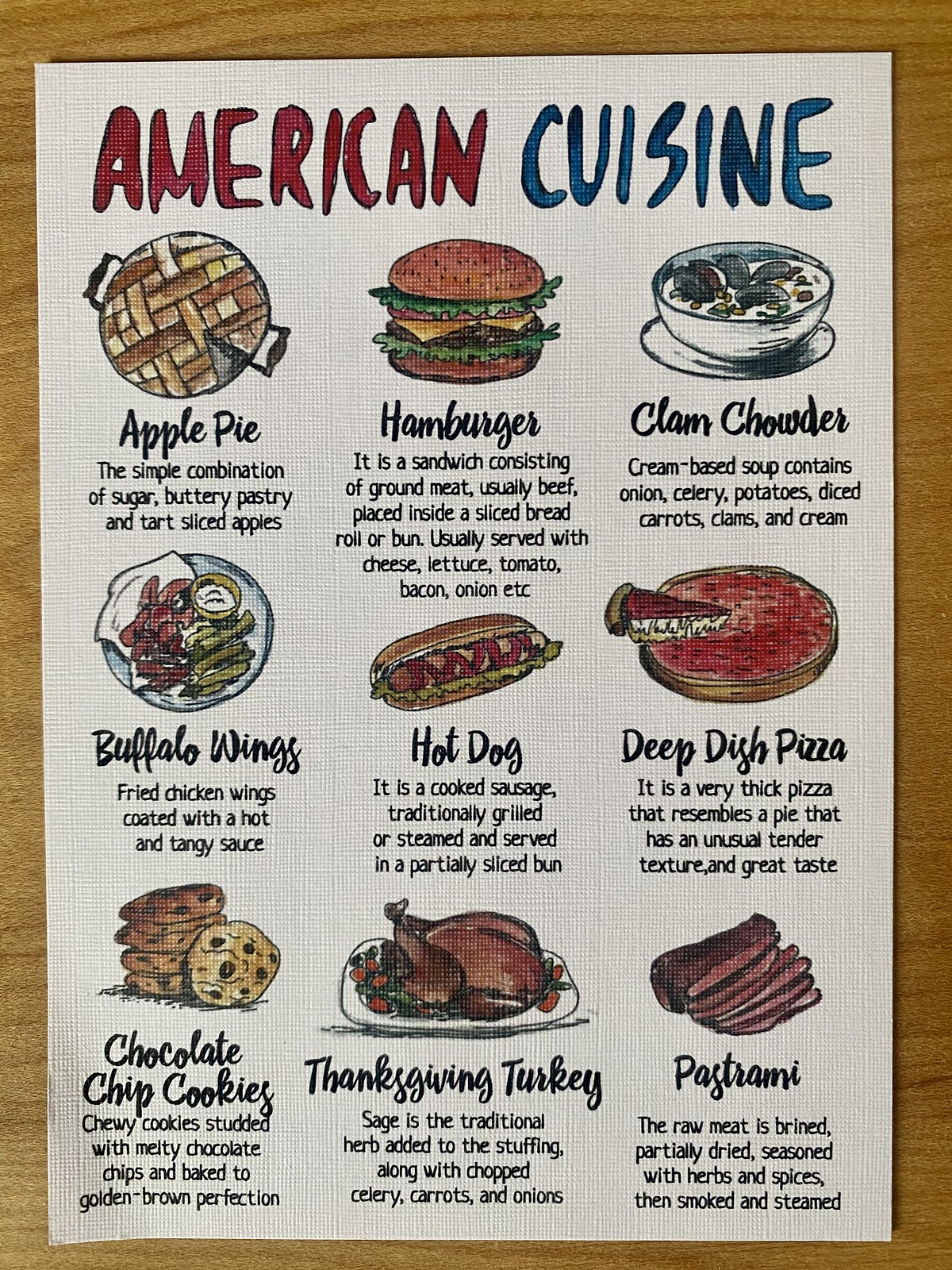This photograph features a meticulously hand-crafted flyer displaying an array of quintessential American cuisine. The flyer is printed on a white linen-textured paper, lending a tactile, refined quality to the piece. It is set against a medium-toned wooden backdrop that further enhances the authenticity and rustic charm of the presentation.

At the very top of the flyer, the title "American Cuisine" is artfully written, with "American" in vibrant red and "Cuisine" in navy blue outlined in black ink, both filled in with a delicate watercolor technique. The entire illustration showcases a skilled hand-drawn aesthetic, emphasizing the care and attention to detail.

Arranged in neat, horizontal rows, the flyer highlights nine iconic American dishes. The top row features:

1. Apple Pie - Detailed as "the simple combination of sugar, buttery pastry, and tart sliced apples."
2. Hamburger
3. Clam Chowder - Described as "a cream-based soup containing onions, celery, potatoes, diced carrots, clams, and cream."

The middle row lists:

4. Buffalo Wings
5. Hot Dog
6. Deep Dish Pizza

The final row showcases:

7. Chocolate Chip Cookies
8. Thanksgiving Turkey
9. Pastrami

Each dish is accompanied by a charming, hand-drawn watercolor illustration and a brief description below, enhancing the flyer’s informative and visually appealing layout.

This detailed and artfully designed flyer not only provides a visual feast but also educates the viewer on the diverse and beloved dishes that comprise American culinary tradition.